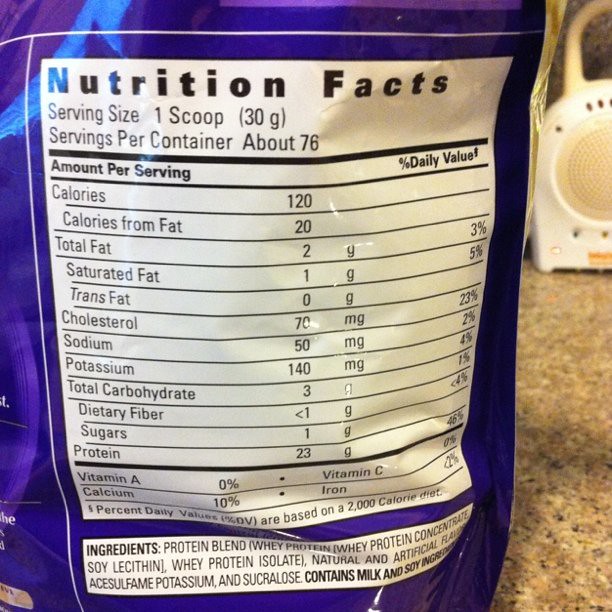The image showcases the nutritional facts and ingredients list on the back of a whey protein supplement package. The package, predominantly blue in color, lies flat on a countertop. The detailed nutritional label, presented in black and white, lists various components such as calories, calories from fat, total fat, saturated fat, trans fat, cholesterol, sodium, potassium, total carbohydrates, dietary fiber, sugars, proteins, vitamin A, vitamin C, calcium, and iron percentages. The ingredients indicate a protein blend consisting of whey protein and whey protein concentrate, with a note specifying the presence of milk and soy ingredients. In the background, there is a device that appears to be a speaker or baby monitor, adding a subtle household context to the scene.